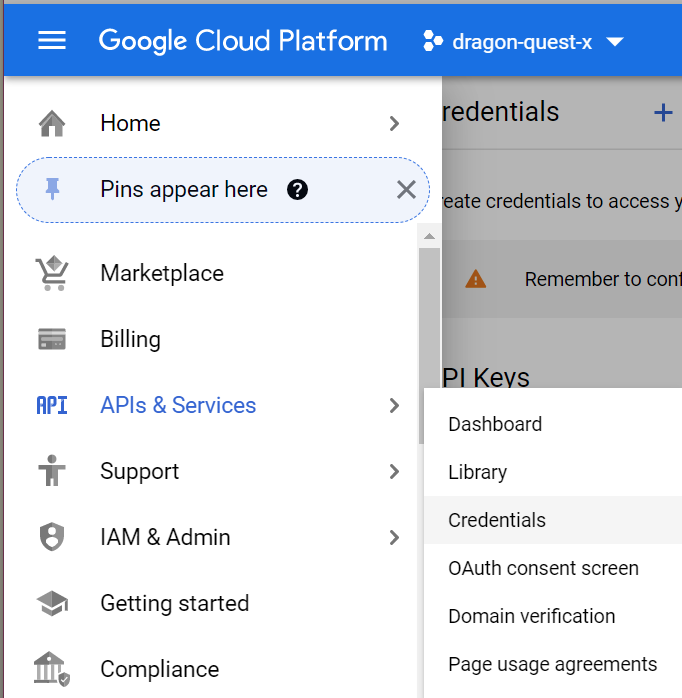A detailed screenshot of a Google Cloud Platform (GCP) dashboard, tailored for managing Dragon Quest X resources. The top of the sidebar prominently displays the "Google Cloud Platform" branding, with "Dragon Quest X" indicated to the right, suggesting this project is specifically configured for handling aspects of the Dragon Quest X game. The sidebar on the left features a variety of tabs for navigating the platform:

- **Home**: Emphasized with a note stating "pins appear here," which likely indicates where users can find commonly used or pinned resources.
- **Marketplace**: For discovering and purchasing third-party cloud solutions.
- **Billing**: To manage and review spending on GCP services.
- **APIs and Services**: For accessing application programming interfaces and various SDKs.
- **Support**: Providing resources and help options.
- **IAM and Admin**: For configuring identity and access management.
- **Getting Started**: Likely offering tutorials or initial setup steps for new users.
- **Compliance**: Tools and resources to ensure adherence to regulatory standards.

Additionally, a separate section on the sidebar includes an options window with the following categories:
- **Dashboard**: Overview of the project's status and recent activity.
- **Library**: Collection of available APIs.
- **Credentials**: For managing authentication and secure access.
- **OAuth Consent Screen**: Settings related to user consent for data access.
- **Domain Verification**: To confirm ownership of domain names associated with the project.
- **Page Usage Agreements**: Details regarding terms and agreements for service use.

The layout is illustrative of the organizational structure and functional navigation offered by GCP for managing cloud-based projects like Dragon Quest X.